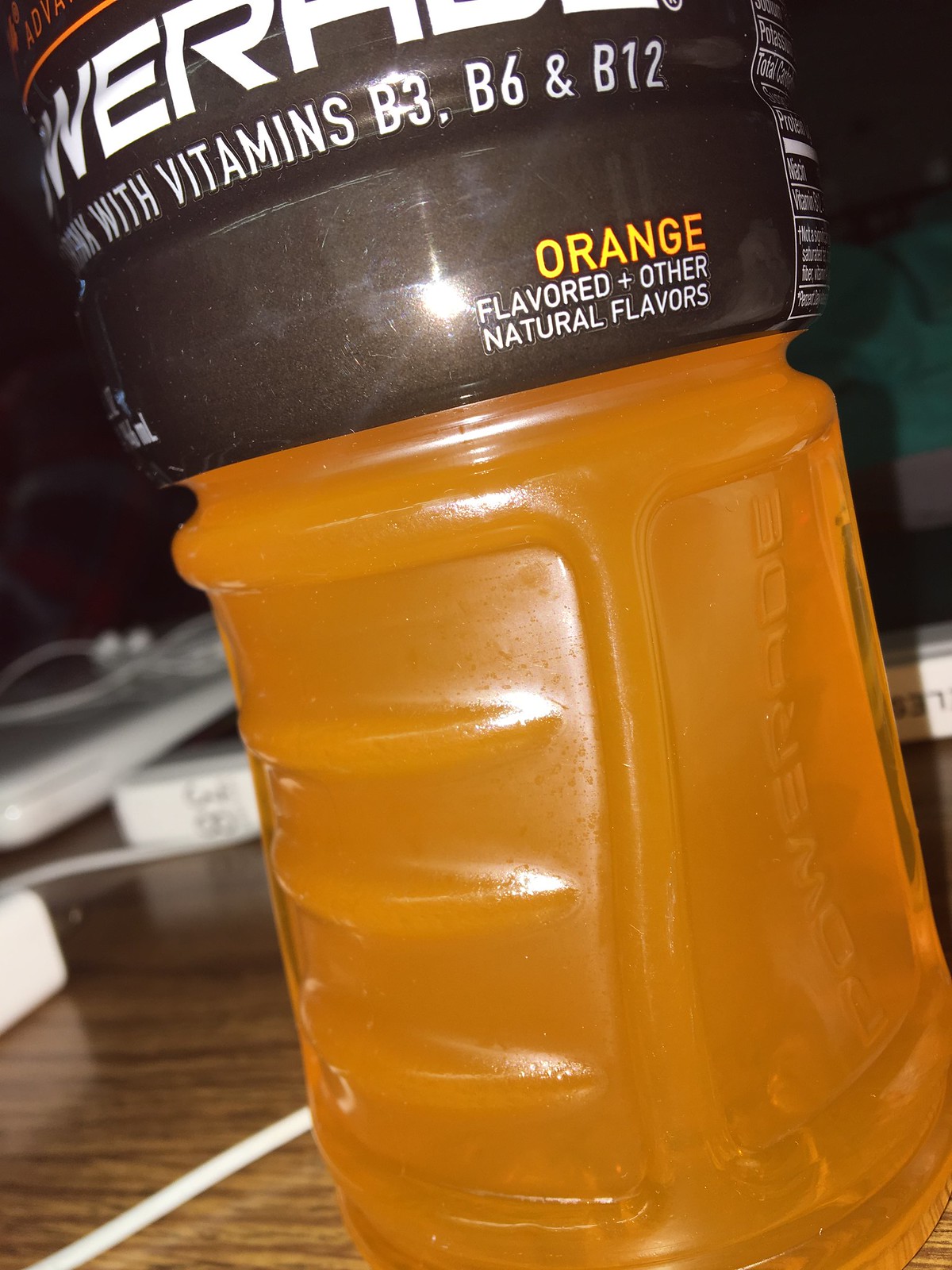The photograph features a clear bottle of orange-flavored Powerade, prominently filled with vibrant orange liquid. The bottle, which has the Powerade logo molded into its side, is adorned with a black plastic label. The label displays the brand name "Powerade" in bold white text and highlights the presence of vitamins B3, B6, and B12. Towards the bottom right corner of the label, the flavor "orange" is indicated in orange text, accompanied by the phrase "flavored plus other natural flavors" in white text. The bottle is placed on a wooden table, partially revealing a nutritional facts label on its right side. In the background, there is a green wall and an assortment of items, including an Apple laptop and an iPod positioned to the left behind the Powerade bottle. This scene appears to be set in a room during the evening hours.